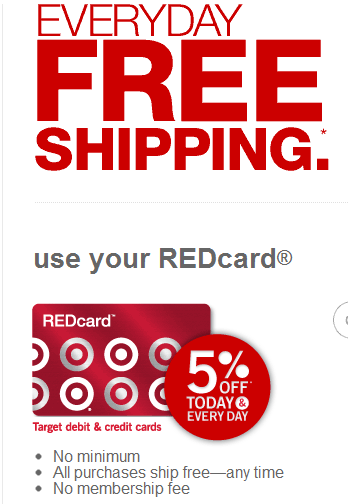**Caption:** 

This advertisement for Red Card, the brand name prominently featured, displays a sleek, minimalist design on a white background with striking red and black text. At the top, the ad captures attention with the phrase, “Every Day” in red text, followed by the compelling title, “Free Shipping,” in larger, bold letters. 

The layout includes ample white space to enhance readability and declutter the presentation. Below, in black font, the text states, “Use Your Red Card.” An image of the card itself is showcased at the bottom, highlighting its distinctive red color. The card features the words "Red Card" at the top and a series of repeating geometric shapes illustrating Target's iconic bullseye logo. These bullseyes, comprised of concentric white and red circles, are arranged in a horizontal row across the card's surface.

Further incentivizing potential cardholders, a circular badge on the advertisement declares, “5% Off Today and Every Day.” Below this, bullet points emphasize key benefits: "No minimum, all purchases ship free anytime," and "No membership fee." The ad clarifies that these benefits apply to both Target debit and credit cards, appealing to a broad audience of shoppers.